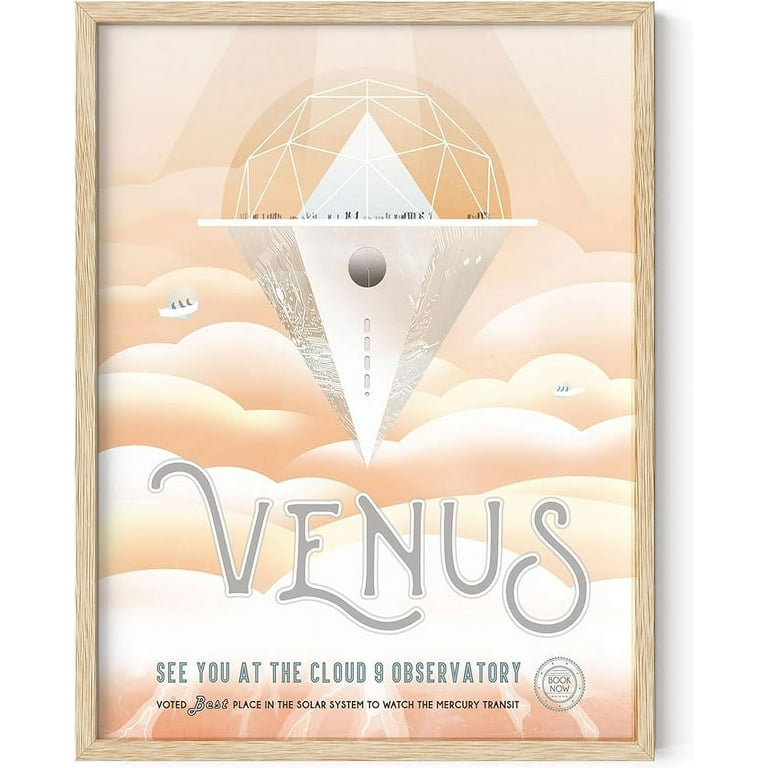The image showcases a rectangular poster oriented vertically, framed by a light beige, raw wooden frame about an inch thick. The poster features a dreamy, fluffy background in hues of pink, peach, light orange, and cream. Central to the artwork is an ice cream cone-shaped structure, capped with a geometrical dome adorned with hexagonal or triangular patterns. Inside this dome, small dark figures stand on a platform. Below, the cone morphs into a series of taupe and cream triangles, culminating in a large dark circle. Fluffy, cotton candy-like clouds envelop the scene, with a small rowboat carrying three people to the left and another, even smaller, white rowboat to the right. At the bottom of the poster, in grey and black text outlined in white, it reads: "Venus. See you at the Cloud Nine Observatory. Voted best place in the solar system to watch the Mercury transit." In the bottom right corner, a circular logo states, "Book now."